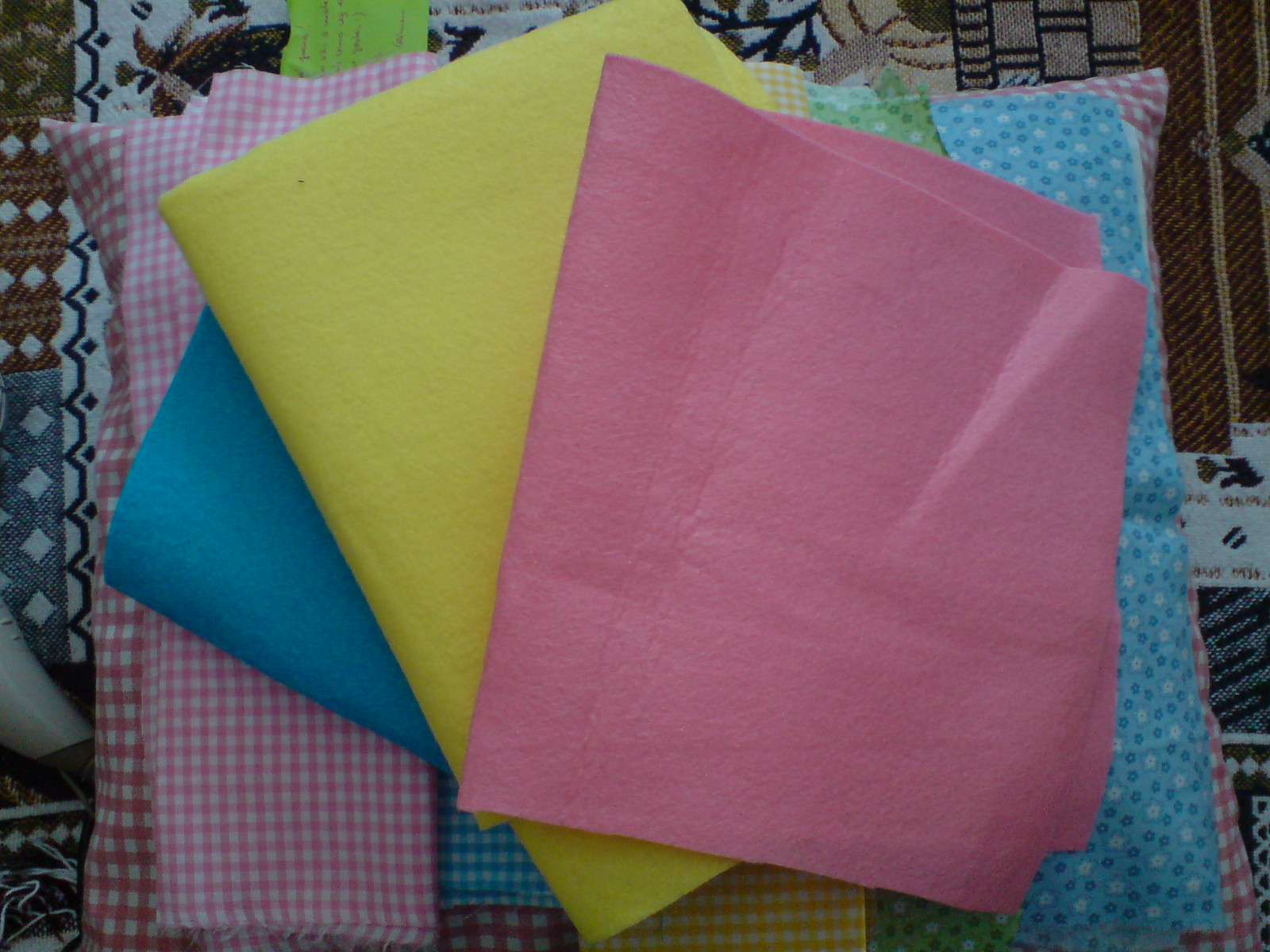This photograph showcases a diverse array of fabric swatches, neatly arranged and set against a richly textured background. At the forefront, there are vibrant, solid-colored cloths: a sky blue, a bright pink, and a cheerful yellow piece of felt. Beneath these, a selection of patterned fabrics unfolds, including a pink and white gingham patchwork, a blue and white checkered pattern, a yellow and white checkered piece, and swatches featuring delicate floral prints in green and blue.

The backdrop of the image provides additional texture and depth, featuring a multi-patterned rug adorned in shades of brown, black, tan, and white. This intricate rug underpins the assortment of fabric swatches and infuses the scene with a tactile richness through its varied textures and raised sections. The carefully folded and layered arrangement of these colorful fabric scraps suggests a readiness for arts and crafts or sewing projects, highlighting both their aesthetic appeal and practical versatility.